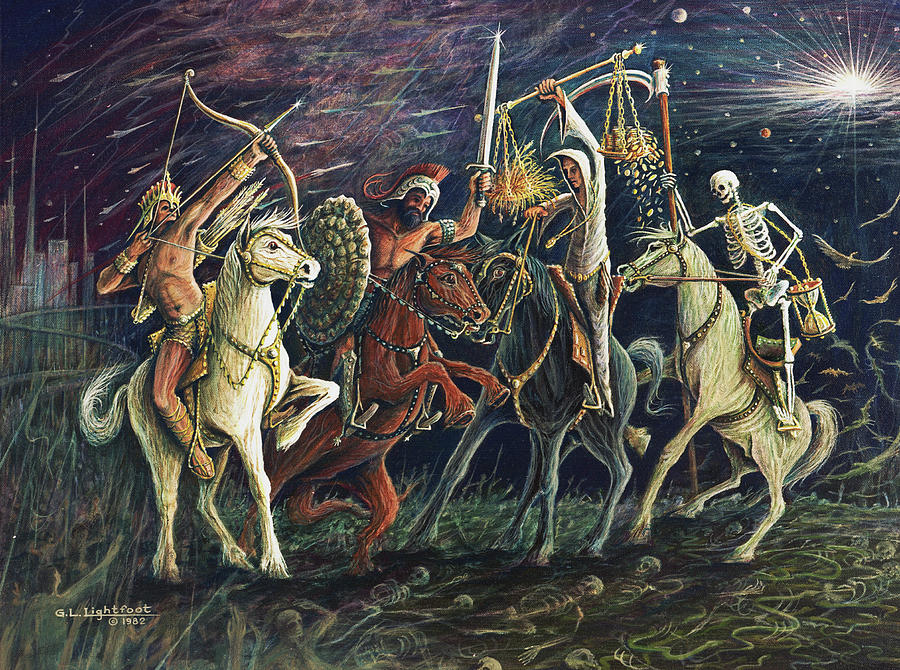The image, signed "GL Lightfoot 1982" in the bottom left corner, is an elaborate oil painting depicting four horsemen dominating the scene. The horsemen, each riding a different colored horse, create a vivid portrayal of what appears to be the Four Horsemen of the Apocalypse. On the far left, a shirtless man wearing a crown and shorts rides a white horse. He is shooting an arrow into the sky, equipped with a quiver full of arrows. To his right, a warrior clad in helmet and armor raises a sword high into the air while riding a brown horse. Next, a figure resembling a wizard, dressed in a cloak and tunic with a necklace, rides a black horse and balances a scale with plants and gold coins, some of which are spilling to the ground. On the far right, a skeleton draped in a satchel-like necklace carrying an hourglass and wielding a sickle rides another white horse.

The backdrop is dark and star-studded, evoking a night scene filled with celestial bodies including stars, planets, and even the universe extending into the top right corner. Arrows fly through the sky, suggesting an ongoing battle. The ground beneath the horsemen is a gruesome field of human skeletons. Adding to the haunting atmosphere, a castle looms in the background on the left.